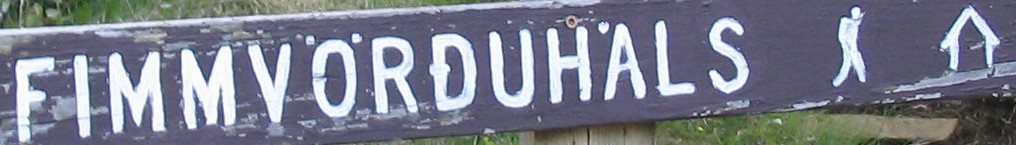This is a close-up photograph of a weathered wooden sign, framed in a thin rectangular format. The edges of the image reveal patches of green grass and light gray areas, suggesting a natural outdoor setting. 

Across the scene is a rectangular piece of wood running from the left-hand side to the upper right-hand side, painted in a tired gray that is chipping on its left side to reveal a lighter gray beneath. The sign features white-painted text on the left that reads "FIMMVORDUHALS." 

To the right of the text, there's a white-painted illustration of a person walking, depicted from a back and slightly right-side perspective. The figure is fully shaded in white, with one leg stepping ahead of the other. Adjacent to this, towards the right, is a simple outline of a house also painted in white, consisting of two vertical lines supporting an upside-down V-shape roof.